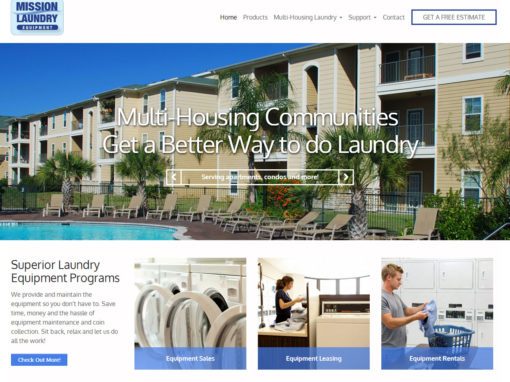The image is a screenshot of a webpage titled "Mission Laundry Equipment." At the top of the page, there are navigation tabs, including Home, Products, Multi-Housing Laundry, Support, Contact, and Get a Free Estimate, with the latter highlighted by a blue box. The background features a scenic pool area with palm trees, expansive apartment buildings, green lawns, various chairs, and trees.

In the foreground, bold text reads, "Multi-Housing Communities Get a Better Way to Do Laundry." Below this, a heading states, "Superior Laundry Equipment Program," followed by a detailed explanation: "We provide and maintain the equipment so you don't have to. Save time, money, and the hassle of equipment maintenance and coin collection. Sit back, relax, and let us do all the work." Directly beneath this text is a prominent blue button labeled "Check Out More."

Further down the page, there are sections highlighting different services. The Equipment Sales section showcases a variety of washers. The Equipment Leasing section features an image of a washing machine in use and a person tending to their laundry. Additionally, the Equipment Rental section displays a blue laundry basket and a person folding a piece of clothing.